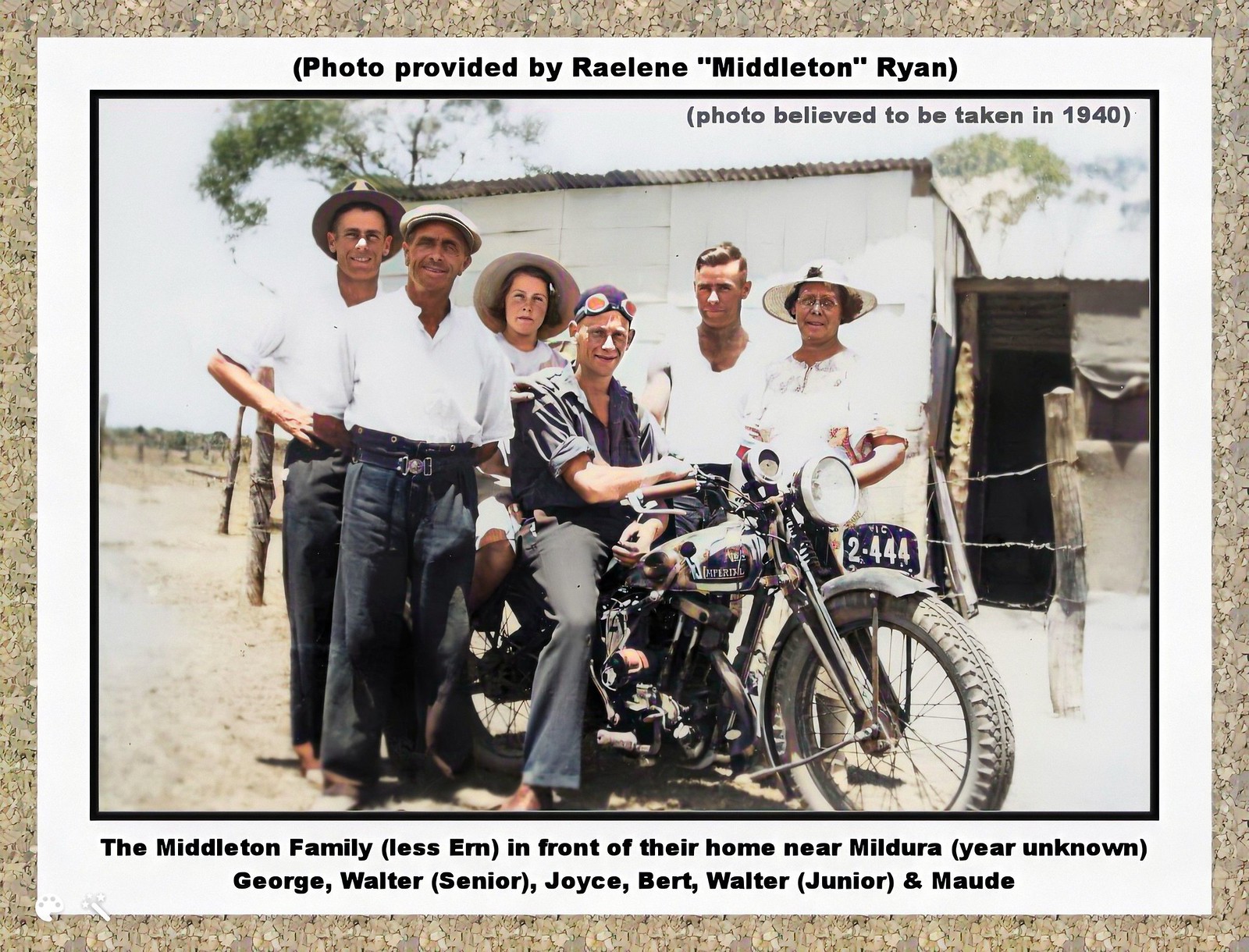The image is a photo bordered by a gray, stone-like cork frame, enclosed by a white border and a thin black line around the actual photo. At the top of the frame, text reads "Photo provided by Raylene Middleton Ryan," and the bottom states, "The Middleton family, less Earn, in front of their home near Mildura, year unknown: George, Walter Sr., Joyce, Bert, Walter Jr., and Maude." The photo captures five people standing around a sixth individual who is seated on a black motorcycle, prominently featuring a license plate that reads 2444. The man on the motorcycle is wearing a black shirt and goggles. The others, two on either side, are mostly dressed in white shirts, with four of them wearing hats. They are positioned on a dirt road in front of a barbed-wire fence and a rundown building with a tin roof, indicating a sunny, likely summer day. The backdrop includes several green-leaved trees, enhancing the rustic charm of the scene.